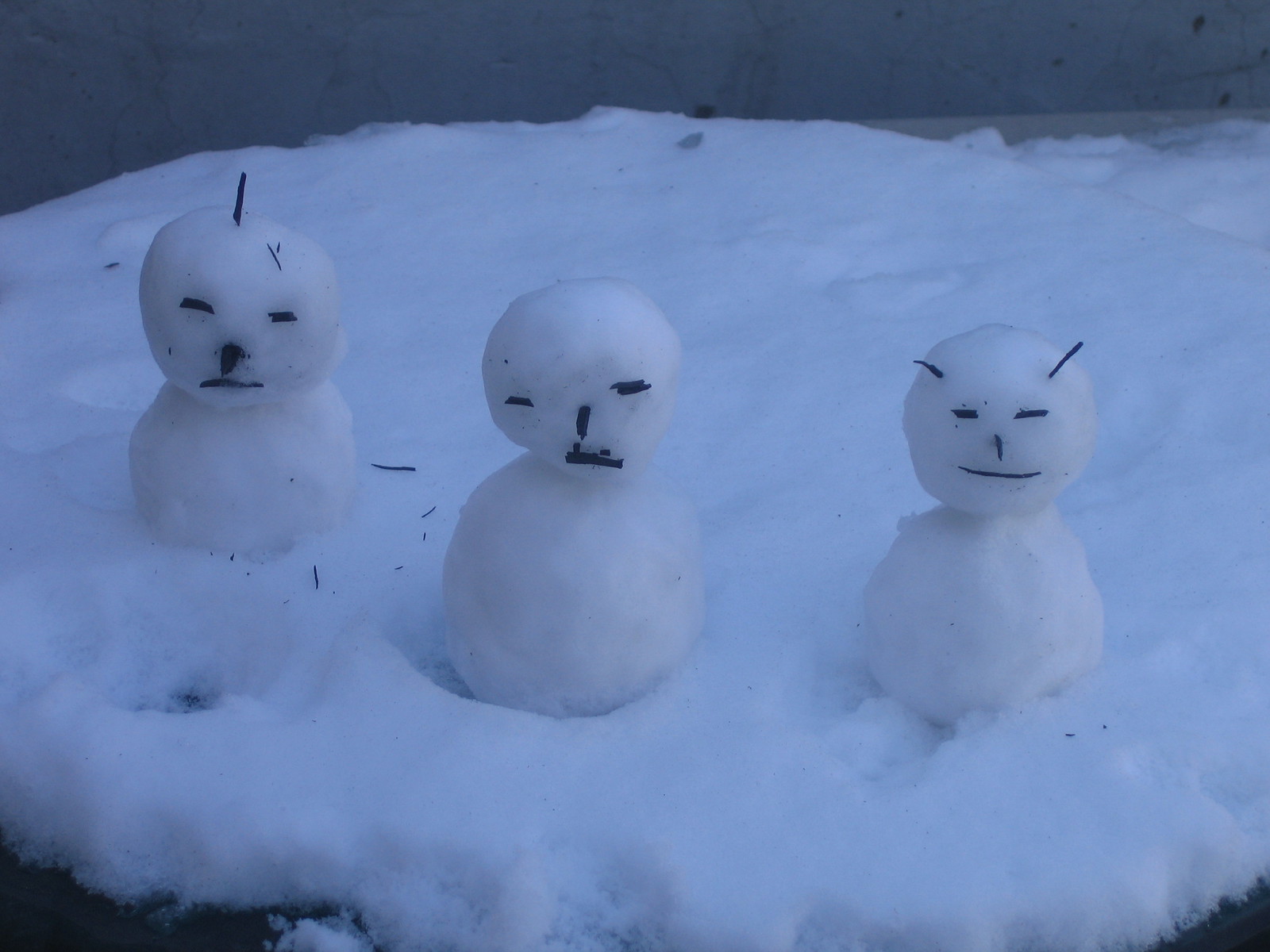This color photograph captures three miniature snowmen arranged on a small patch of snow. Each snowman consists of a small snowball for the body and a smaller snowball for the head. The snowmen are crafted with fine, splinter-sized sticks serving as their facial features. The snowman on the left sports a twig sticking up from its head, slanted eyes made from vertical sticks, a pointy black stick for a nose, and a horizontal stick for a mouth. The middle snowman has the simplest design, with two short horizontal sticks for eyes, a stick for the nose, and a horizontal mouth. The snowman on the right features two little twigs resembling antennas on top of its head, horizontal sticks for eyes, a stick for a nose, and a slightly curved thin stick for a mouth, creating a subtle smile.